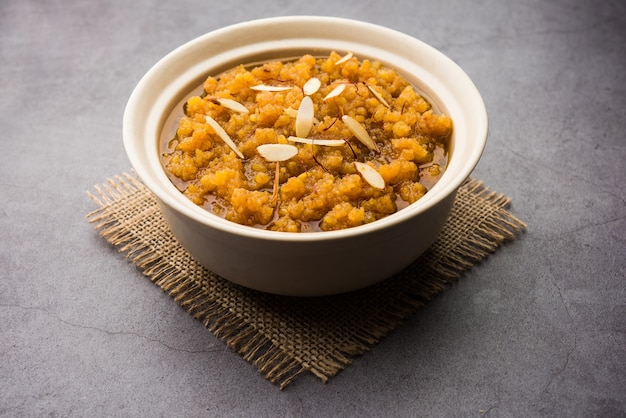In this detailed image, a round, white porcelain bowl sits atop a small, square placemat made of tan burlap with fringed edges, resembling a rustic doily. The bowl, somewhat deep and cream-colored, is filled with an amber, bumpy-textured substance that appears to be mashed squash. Finely sliced white almonds are scattered on top, adding a decorative and nutty touch to the dish. This setup is arranged on a light gray hard surface, possibly granite or concrete, enhancing the natural and wholesome aesthetic. No utensils are present, suggesting this is a meticulous presentation piece.